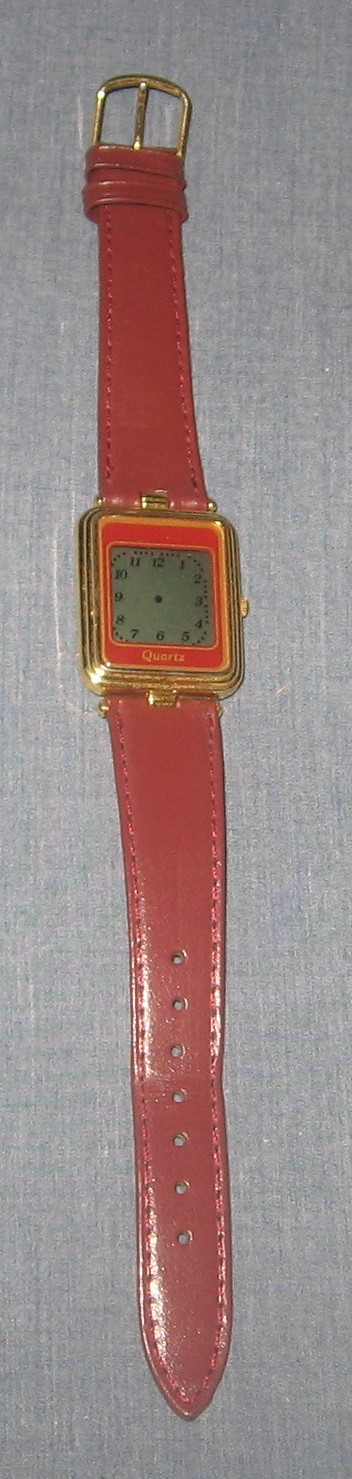This color photograph features a close-up of an analog wristwatch laid out vertically, with the entire watch band and face displayed in a narrow frame. The background is a light slate gray, providing a subtle contrast to the striking red watch band, which appears to be made of either red vinyl or red leather. The watch face is square and encased in a gold or gold-plated metal frame, encompassing an inner square of what looks like red enamel. The dial of the watch is medium to dark gray, adorned with black Roman numerals. Although the hands of the watch are not visible, possibly due to the lighting or their diminutive size, the overall aesthetic is both bold and elegant.